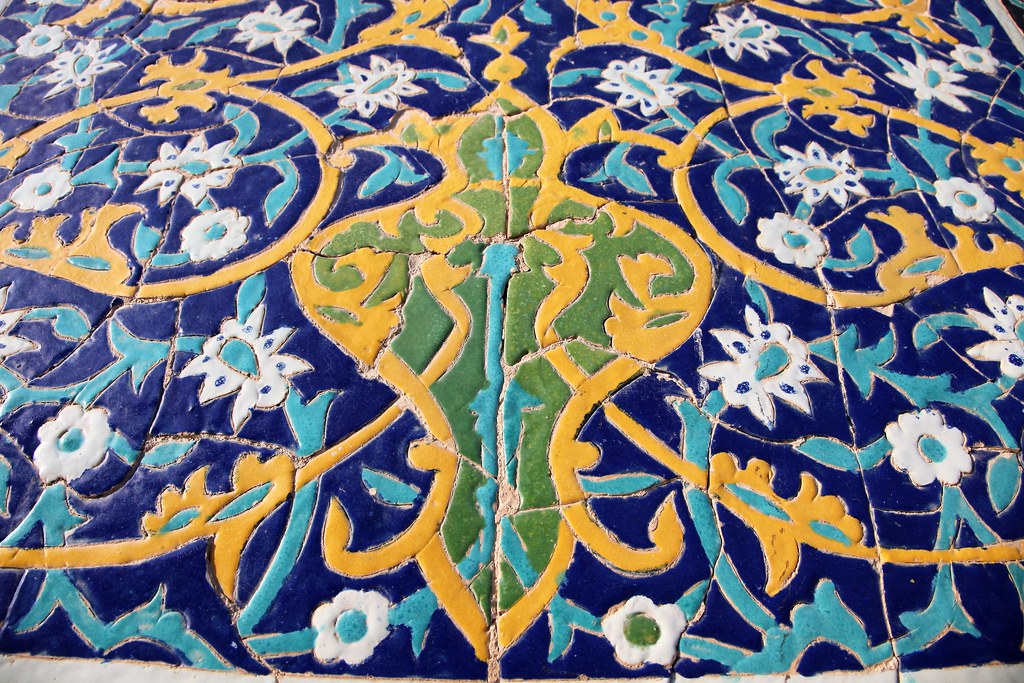This image showcases a detailed close-up of a vibrant, three-dimensional, tile mosaic adorned with a myriad of intricate, textured shapes. The centerpiece of the mosaic features a curvy, spear-like symbol outlined in yellow, filled with patches of lime green and baby blue, while surrounded by dark blue segments. Encircling this central design are intertwined blue vines bearing delicate white flowers, each petal intricately speckled with light blue. Interspersed among these blue vines are golden vines with associated golden flowers, adding a layer of richness to the overall design. The tiles, reminiscent of Mediterranean art, create a visually arresting pattern predominantly composed of white, dark blue, light blue, yellow, and green hues. The surface, riddled with numerous cracks, adds character and a sense of age to the piece. Despite its ambiguity regarding whether it adorns a floor or a wall, the lack of contextual clues or text in the image only heightens its enigmatic beauty.